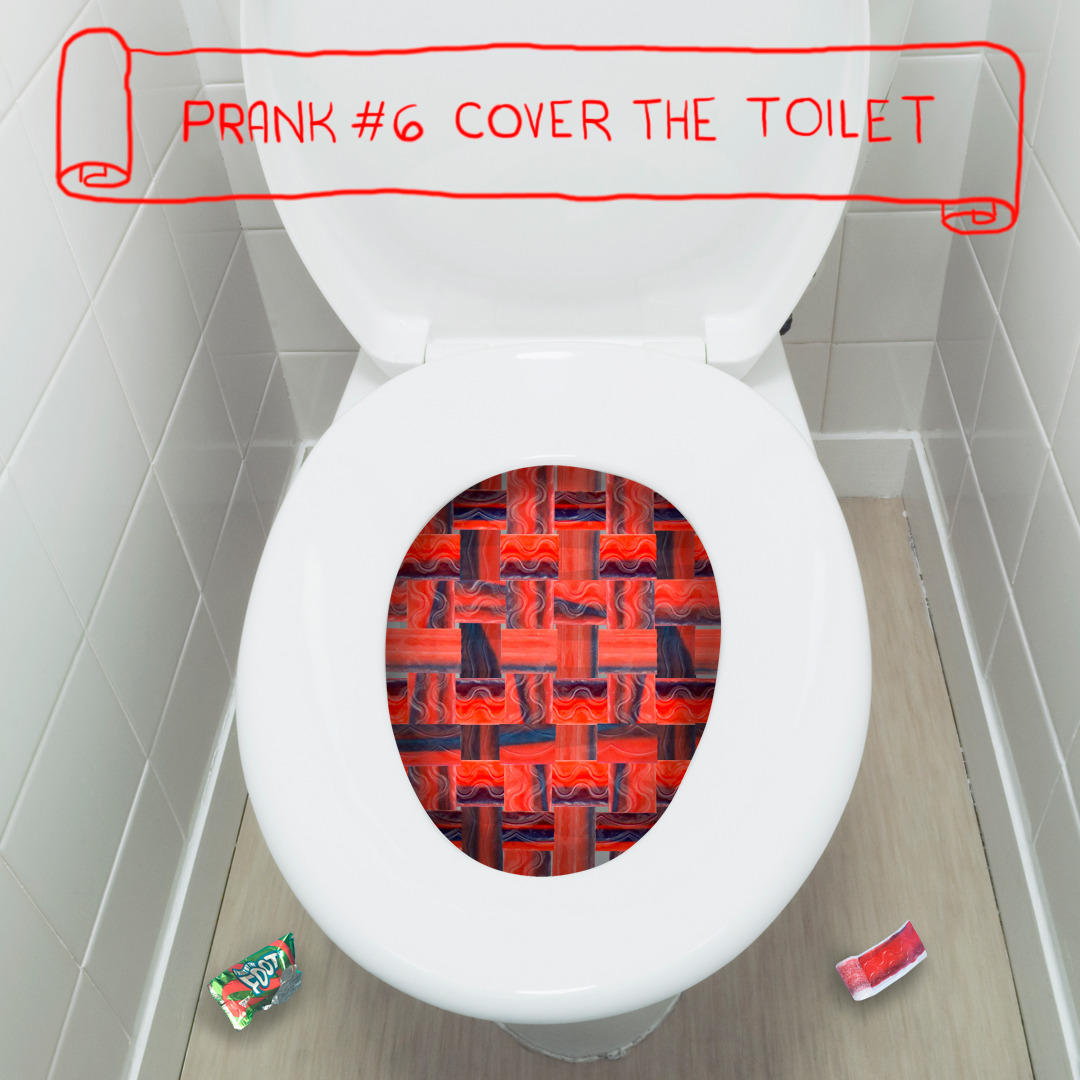This image showcases a prank, labeled in red text as "Prank Number 6: Cover the Toilet," edited onto the picture near the top of the toilet tank. The scene is set in a very small stall adorned with white walls and a light grayish or tan wood floor. At the center of the image is an open, white toilet, whose bowl is intricately covered with unwound rolls of red and black Fruit by the Foot, resembling the latticework on an apple pie. The dedication to the prank is evident with the Fruit by the Foot meticulously arranged to cover the entire opening, effectively making any use of the toilet impractical. Scattered on the floor are bits of trash, including remnants of the Fruit by the Foot wrappers, adding to the prank’s chaotic humor.